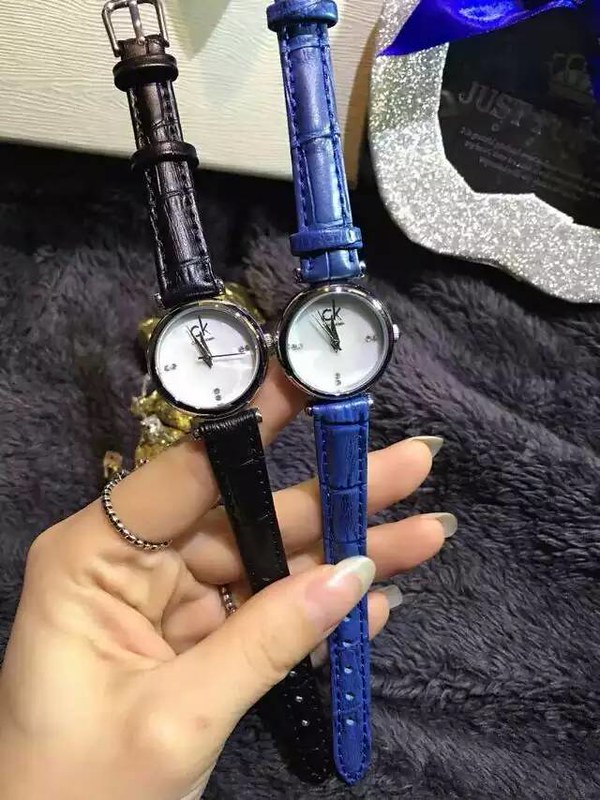In the image, two identical Calvin Klein (CK) watches, set to the exact same time, are prominently displayed. Each watch features a snakeskin strap, with one in a vibrant blue hue and the other in a sleek black shade. A woman’s hand elegantly holds the watches, revealing her unpolished nails adorned with a ring on her pointer finger and another on her ring finger. The watches are positioned over a luxurious black fur blanket. Beside the blanket, there is an intriguing silver object that might be a hat with a silver trim, partly covering a blue flag design against the backdrop of a white wall.